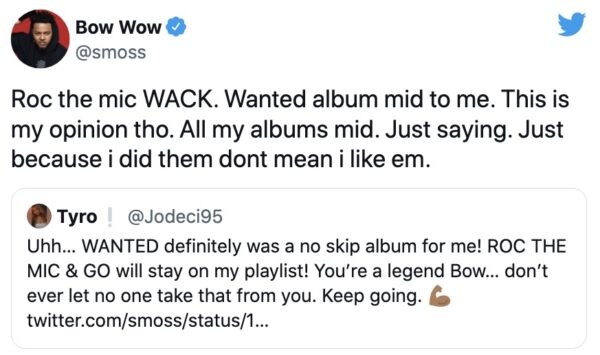The image depicts a Twitter conversation between Bow Wow (@Smoss) and Tyro (@Jodeci95). Bow Wow, identified as a Black man, shares a candid opinion about his music career, stating:

"Rock the Mic was whack. Wanted album was mid to me. This is my opinion though—all my albums are mid, just saying. Just because I did them, doesn't mean I like them."

Key terms are abbreviated or slang, such as 'Rock' spelled "R-O-C," 'Mic' for microphone, 'Whack' in all capitals "W-A-C-K," and 'Mid,' meaning mediocre. Bow Wow also abbreviates 'though' as "C-H-O" and 'them' as "'E-M" without proper punctuation.

Tyro responds supportively, saying:

"Wanted was definitely a no-skip album for me! Rock the Mic and Go will stay on my playlist. You're a legend, Bow. Don’t ever let anyone take that from you. Keep going 💪."

Tyro’s message praises Bow Wow’s work, emphasizing specific tracks like “Rock the Mic” and affirming his legendary status in the music industry. The Twitter URL in the post header is partially obscured.